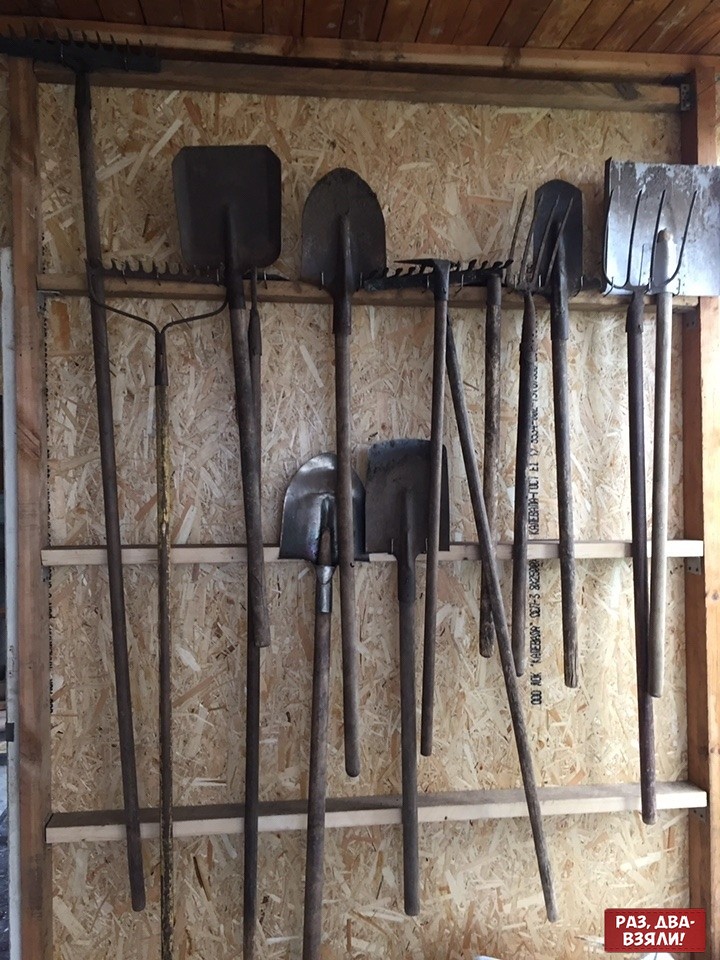The photograph depicts the interior of a rustic, possibly unfinished, barn or garage with wooden walls and framing. The top part of the image shows the roof, constructed of wooden planks and floorboards, with a visible rectangular frame structure. From the top beam hang a variety of weathered yard tools; on the far left is a long-handled rake. The next beam below holds garden implements arranged from left to right: another rake, a square-headed shovel, a hoe, a round-headed shovel, another rake, an additional garden tool, a forked shovel with tines, another shovel, and a fork-like tool with a long handle, culminating in a very square-headed shovel. 

Central to the image, on the lower beam, there are two more shovels side by side, one with a square head and the other with a rounded head. These tools are described as black, rusted, and well-worn, some handles darkened and greasy from use. They appear to be affixed to the wall with nails. The wall itself is unfinished, either floorboard-like wood or fiberboard, adding to the rustic ambiance. In the bottom right corner of the image, there is a small red rectangle featuring white letters in a foreign script, partially legible as "P A 3, A B A - B (backwards B) 3 (backwards R) A (without the slash in the middle) N !". The photograph is portrait-oriented and focuses primarily on the array of worn handling tools against the light wooden background.